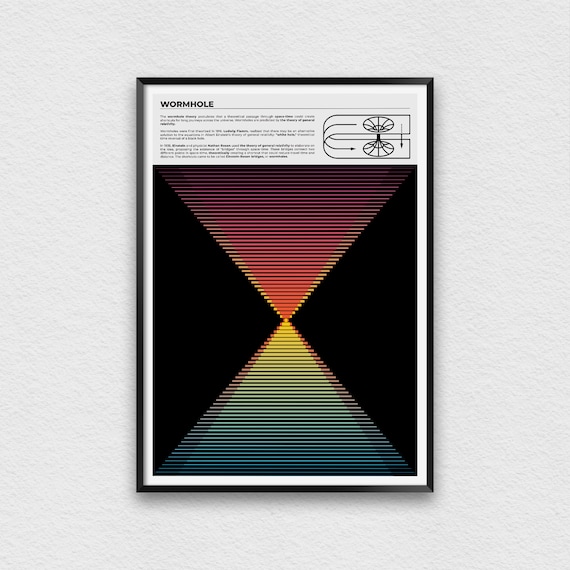The image depicts a framed artwork set against a white, paper-like textured wall. The central piece is a poster with the title "Wormhole" written in black against a light gray background, positioned at the top right of the frame. Below the title, a thin black line separates it from three paragraphs of text that are too small to read. On the left side of the text, there is a black-on-white ink drawing illustrating a wormhole as two upside-down funnels connected at their narrow ends. Beneath this drawing is a black rectangle containing an intricate diagram. This diagram features two triangles touching at their tips, forming an hourglass shape. The upper triangle has lines transitioning from deep red to orange, while the lower triangle's lines change from yellow at the top to green and blue towards the tip. The artwork visually and textually conveys the concept of a wormhole as a shortcut through space, drawing parallels to explanations found in science fiction and scientific discourse.